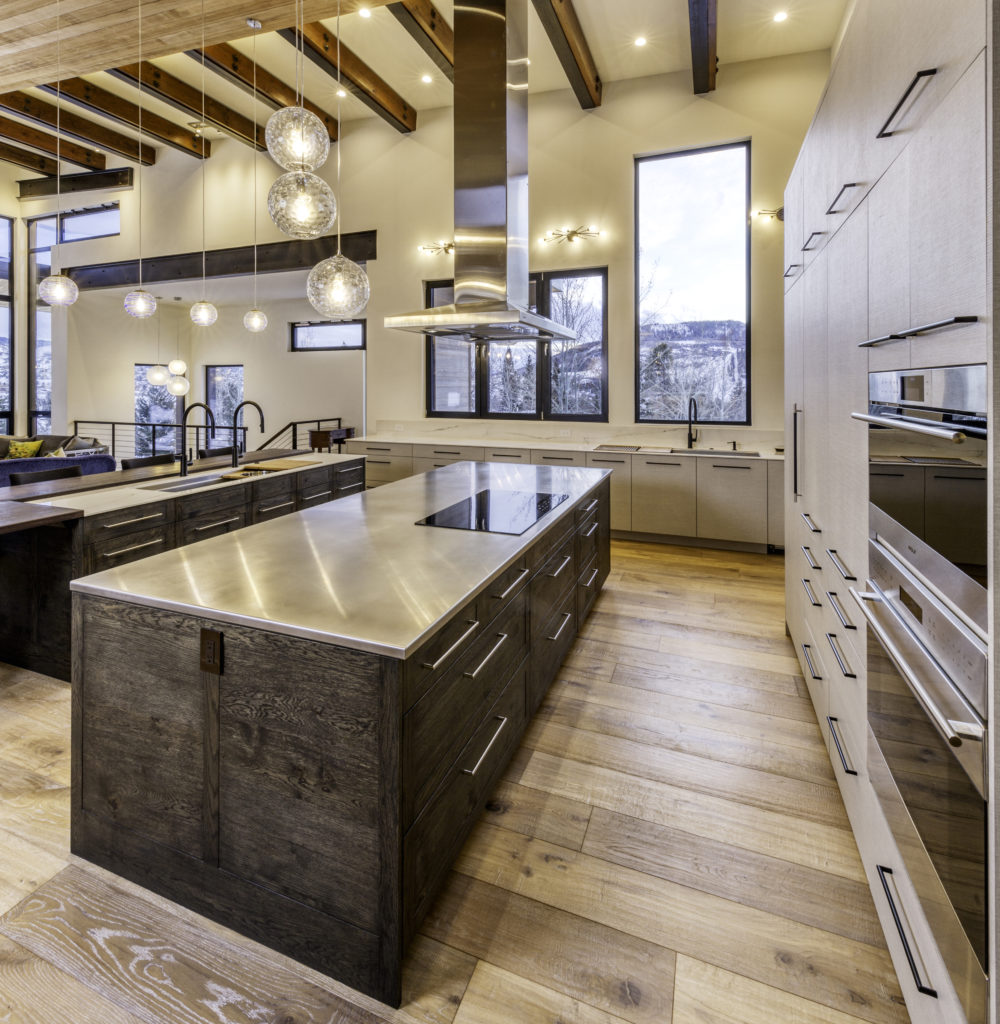The image depicts an expansive, modern kitchen characterized by its spacious layout and multiple functional areas. The room features a hardwood floor and a beige ceiling accented with prominent brown beams. Central to the kitchen are several islands equipped with silver-surfaced cabinets, each adorned with sleek silver handles and pull-out drawers. A notable feature is the black, square-shaped ovens integrated into the cabinetry. On the right side of the image, more cabinets and a couple of pull-out ovens are visible.

Large windows on the back wall allow natural light to flood the space, providing a glimpse of the outdoors. There is an additional large window to the right, positioned above a sink with a black faucet. The ceiling, which also houses lit white lights, appears white under these lights. The overall layout, including multiple sinks and the central counter with an oven and overhead hood, suggests that the kitchen could be well-suited for activities such as cooking classes. This very large kitchen combines functional design with a modern aesthetic, making it an ideal space for culinary endeavors.